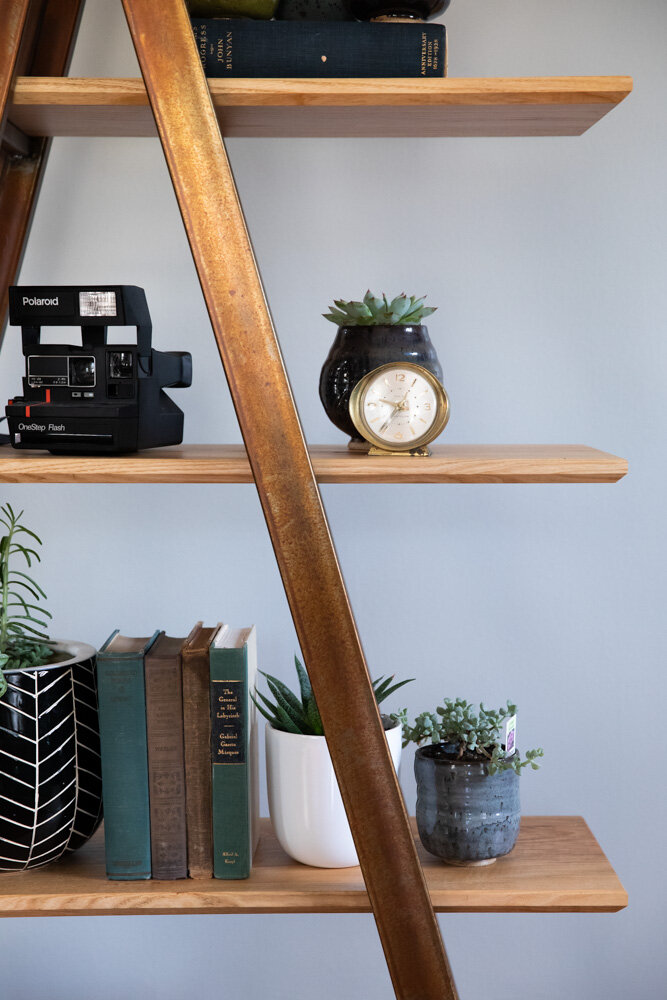The image depicts a wooden ladder-style shelf unit with three visible shelves set against a gray wall, incorporating a unique vertical wooden piece as part of its design. The bottom shelf hosts a variety of items, including four old-looking books flanked by an assortment of potted plants. Specifically, there is a large pot with a black chevron pattern containing a green plant, a white ceramic pot with a succulent, and a smaller blue-gray pot with a green plant and an unreadable tag. The middle shelf features a vintage black Polaroid camera and a gold-framed clock doubling as a planter, holding a succulent in a ceramic pot. The top shelf, partially obscured in the image, displays a lone large blue book and what appears to be additional ceramic pots atop it. Each shelf is thoughtfully arranged, contributing to a balanced and aesthetically pleasing composition.